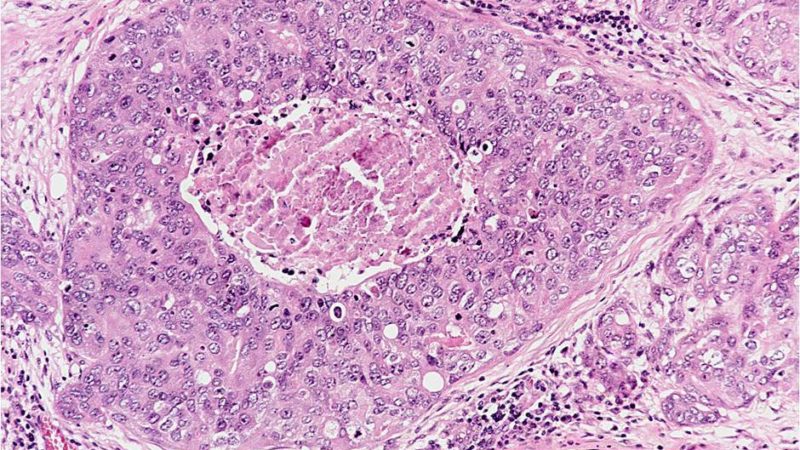The image depicts a microscopic close-up of biological tissue, most likely cells, on a rectangular slide. The background is predominantly pink, with various purple and white specks that suggest cell walls or organelles like mitochondria. Centrally, a prominent, circular mass with a white outline is visible, resembling a wrinkly, brain-like structure, darker in the middle. This central mass is surrounded by an oblong, pinkish-purple region filled with tiny circles or dots in shades of white and darker purple. On the left side, there are more of these pinkish-purple and white circles, while the right side features a stream of white with scattered purple dots. The right-bottom corner continues this pattern with purples and pinks. Overall, the image strongly resembles what one might observe when looking at tissue samples stained with dye under a microscope, with elements resembling blood cells or platelets scattered throughout.